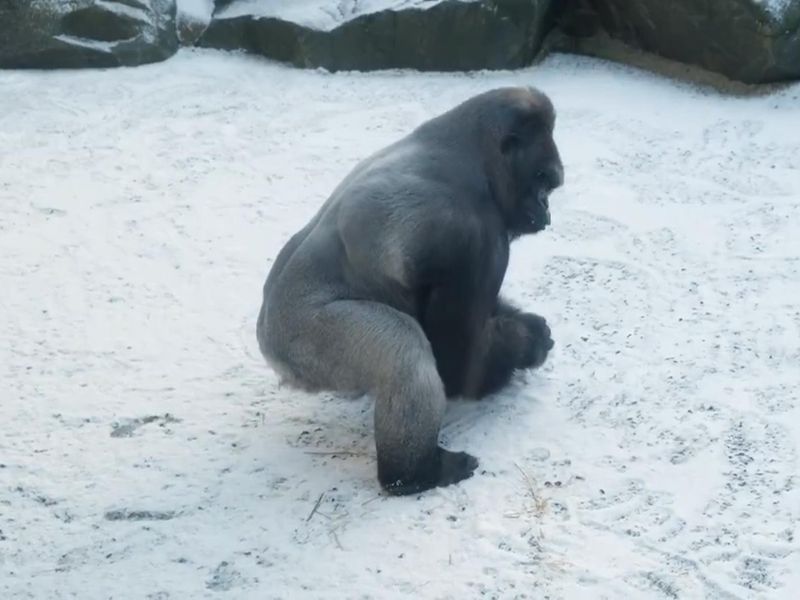The photograph captures a black gorilla squatting on a snowy, flat ground, with bits of grass peeking through the snow. The gorilla, sparsely marked with gray or white fur on its knees, back, and shoulder, appears to be beating its hands on the ground. The image angles slightly downward, providing a perspective just above the gorilla's height. The background showcases large, dark gray rocks with patches of snow atop them. The gorilla, with its large humped head, prominent muscular arms, short legs, and small yet wide feet, stands out as the main focal point of this stark, outdoor scene.